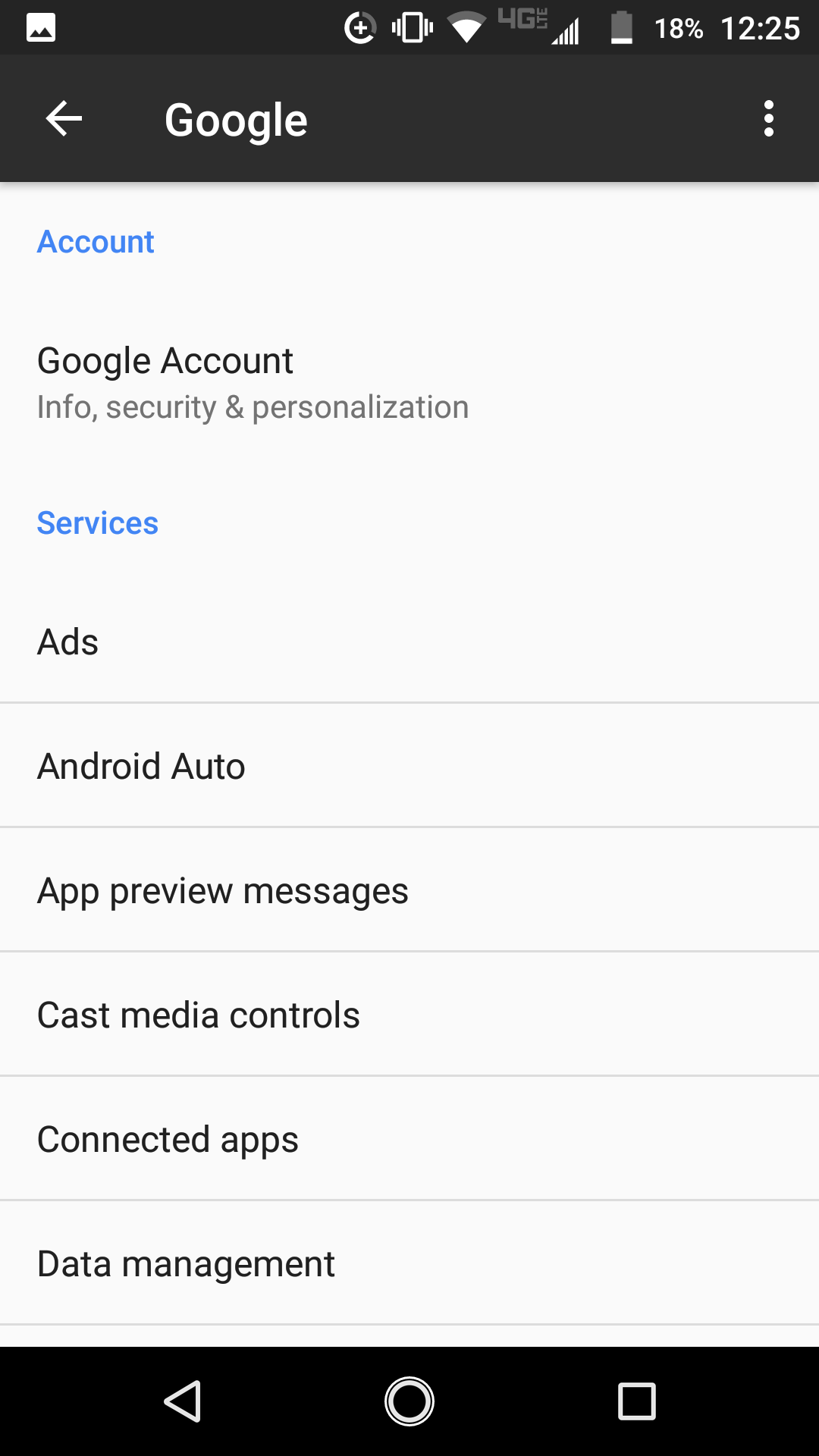The image depicts a screenshot of the settings section of a Google account on a mobile device. At the top, the word "Google" is prominently displayed, followed by the word "Account" in blue text just beneath it. Directly below, "Google Account" serves as a header, introducing the sections titled "Info, Security, and Personalization."

Further down, also in blue text, is a section labeled "Services." Under this category, various subsections are listed, which include "Ads," "Android Auto," "App Preview Messages," "Cast Media Controls," "Connected Apps," and "Data Management." These subsections are organized vertically, making it easy to navigate.

At the bottom center of the screenshot, a circular button is visible, likely indicating the home button. To the right of the circular button, there is a square button, which is typically used for showing recent apps. To the left, a triangle button pointing to the left can be seen, which usually functions as a back button on Android devices. This comprehensive view provides users with quick access to manage different aspects of their Google account settings.